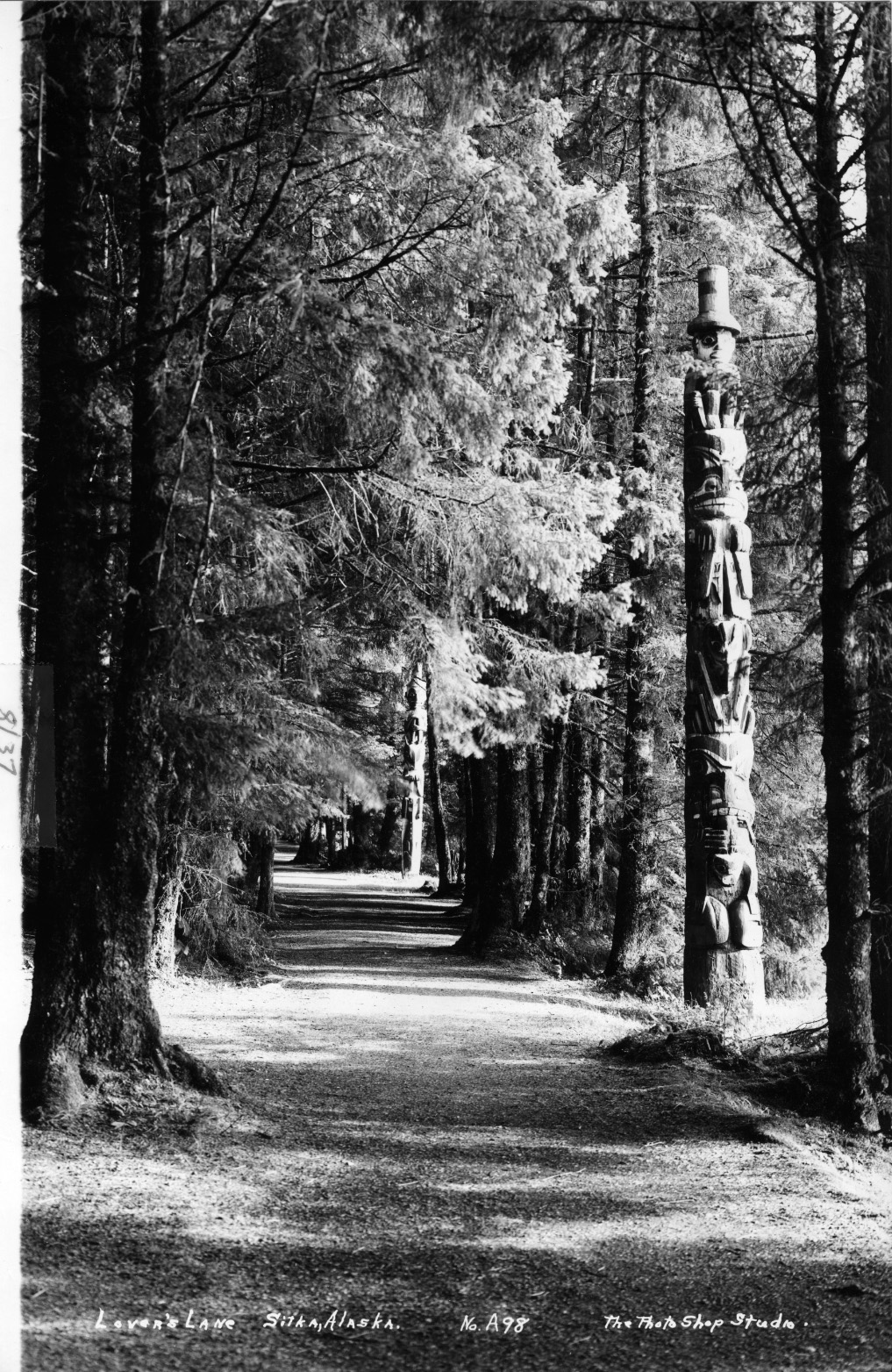This black-and-white photograph, labeled "Lovers Lane, Sitka, Alaska, number A98, The Photoshop Studio," captures a serene, wooded trail. The narrow, dirt pathway stretches through a dense forest, bordered by tall trees rich with leaves. Sunlight filters through the canopy, casting dappled light and shadows on both the trail and the surrounding foliage. Dominating the right side of the scene is a striking totem pole adorned with various carved faces, the topmost figure sporting a top hat. The detailed craftsmanship of the totem pole contrasts with the natural beauty of the trees and the forest path, creating a harmonious blend of natural and cultural elements. The bottom right border of the photograph indicates it is part of a series, marked as '8 out of 37'.